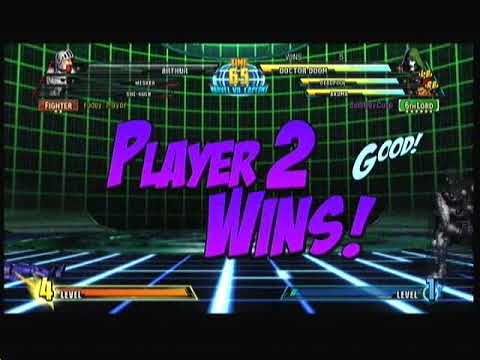This screenshot captures the intense action from a 3D fighting video game set atop a cityscape featuring multiple skyscrapers and buildings. Key elements include four health bars marked in green and yellow hues indicating character vitality. On the far right, a character in a black trench coat stands ready, juxtaposed by an airborne opponent engaging in combat. Above the fray, a maroon helicopter hovers, adding dynamic tension to the scene. At the bottom, distinct level indicators mark the gaming progress: "2 level" in bright green on the left and "level 5" in orange on the right. A backdrop banner reads "Daily BL something," suggesting in-game lore or a contextual element. Additional details like scaffolding, railings, and wisps of smoke further enhance the immersive urban rooftop fight setting, reminiscent of classic arcade fighting games.